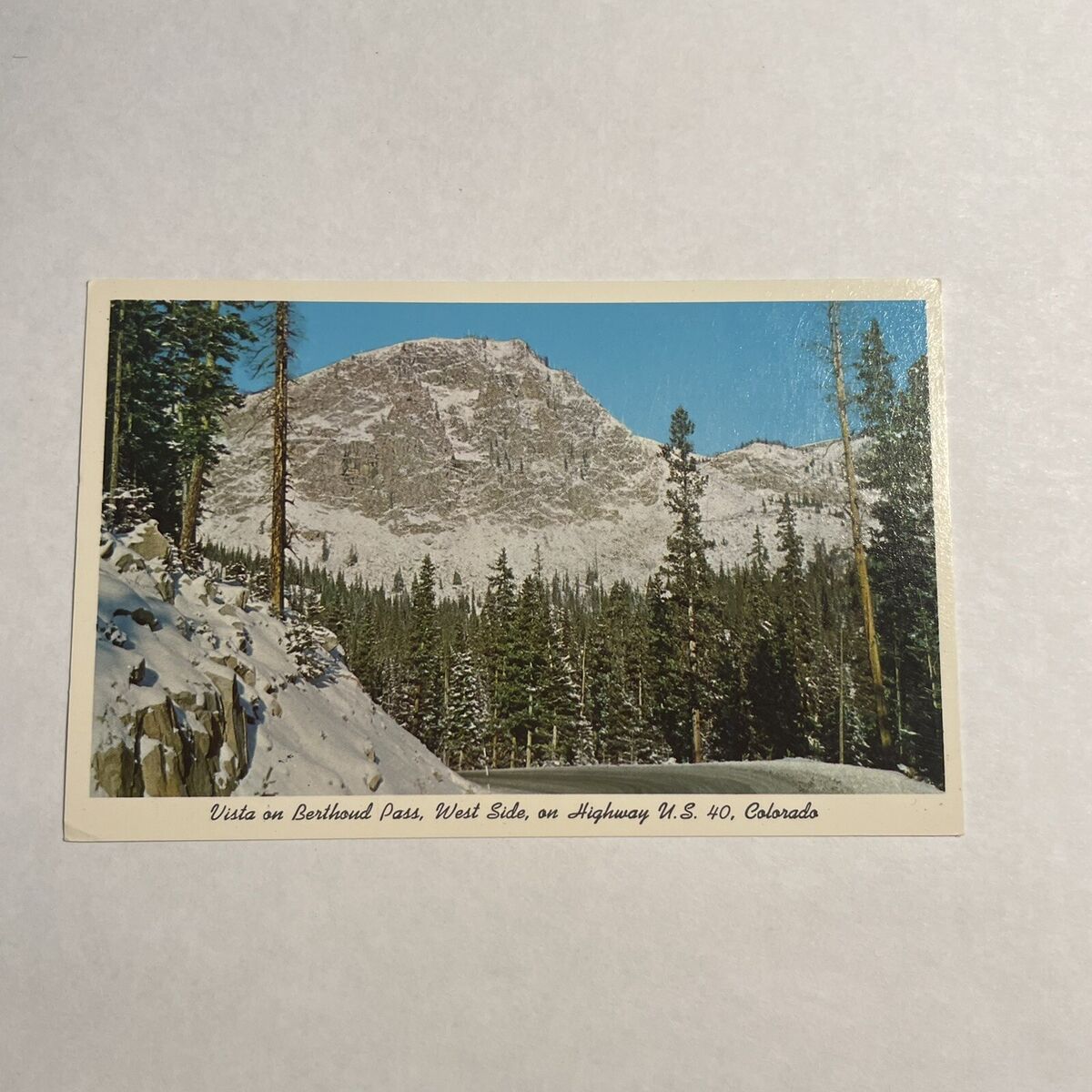The image shows a photograph of a vintage postcard set against a white-grayish background. The postcard itself is bordered by a half-inch white margin, slightly yellowed with age, which adds to its vintage charm. The main subject of the postcard is a picturesque vista of the Berthoud Pass on the west side of Highway US-40 in Colorado. Dominated by snow-capped mountains and dense green evergreen trees, the image highlights a serene, frosty forest scene. The highway, partially visible and bordered by snowbanks, curves through the landscape, enhancing the sense of depth and natural beauty. The text at the bottom clearly reads, "Vista on Berthoud Pass, West Side on Highway US-40, Colorado," providing context to the stunning view captured in the center of the postcard.